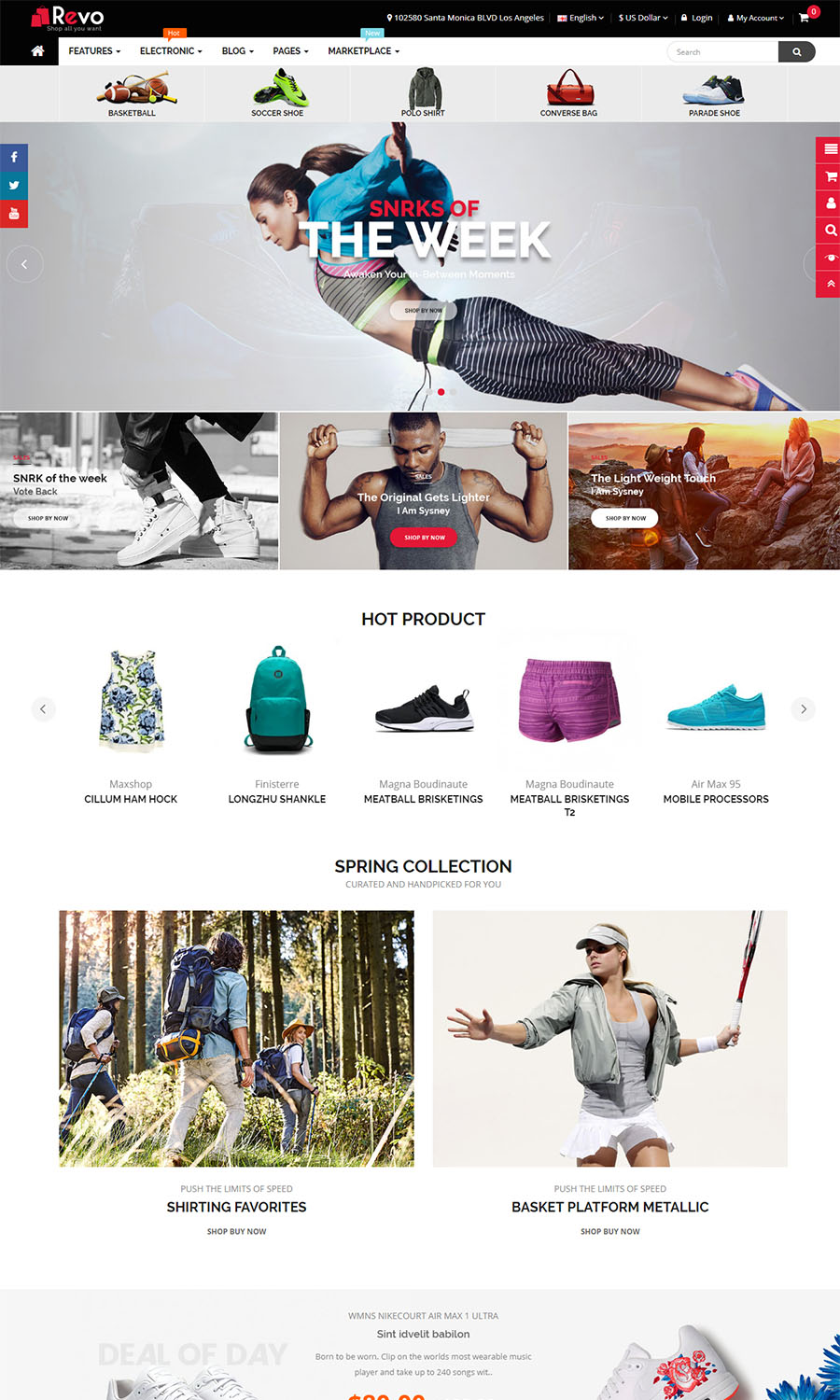Front and center, a digital display featuring "The Week" is prominently shown with the top portion displaying the logo "Revo." Surrounding the main text are various gear and accessories including shoes, bags such as backpacks and purses. On the left side of the image, social media icons, notably Facebook in blue and Reddit in red, are visible. On the far right, an array of red squares with white centers is displayed, with the text "In Our Case of The Week." 

In the middle of the scene, a person, possibly stretching with arms extended forward, is partially visible wearing a grey tank top and draping a white towel over their back. Behind this individual, there are people engaged in hiking, highlighting the outdoor and active theme of the display. Additional items include a green backpack, black shoes, purple shorts, and a blue shoe, emphasizing a range of athletic apparel and accessories. The background features a grey color scheme to accentuate the vibrant products and a nod to an athletic brand, reinforcing the active lifestyle promoted.